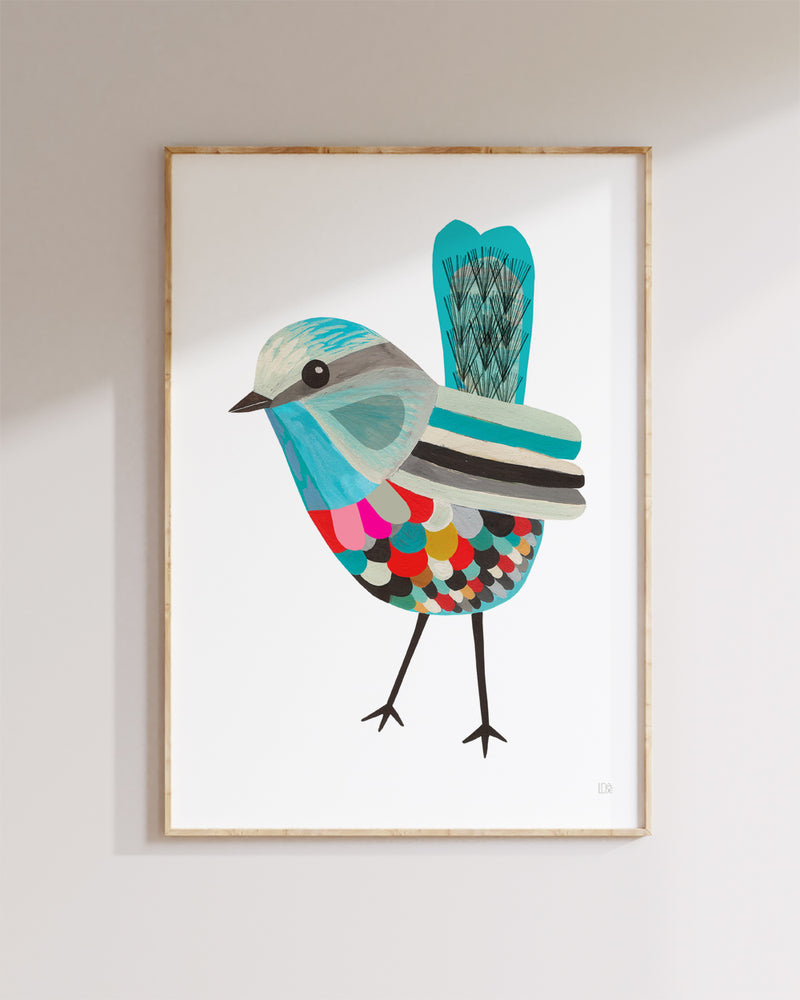This photograph captures a vertically aligned, framed image of a vividly painted bird, possibly a watercolor or a computerized version, hanging on a plain white wall. The frame is a thin, light-colored wood with some darker brown knots. The light illuminates about three-quarters of the picture, leaving the remainder in shadow, hinting at a possible shelf underneath.

The bird itself stands upright with a turquoise-blue, white, and gray head. A dark gray stripe stretches across its black eye. Below its beak, the bird's face is adorned with patches of blue and gray. Its wings display stripes of blue, white, black, and gray, and the tail is predominantly blue with fine black lines. The bird's legs and short beak are black.

The bird's chest and underbelly are a colorful mosaic of overlapping circles in shades of red, pink, light pink, dark pink, gray, blue, black, yellow, turquoise, green, and even gold. The painting is signed in the lower right corner with what appears to be the artist's initials, possibly "ER."